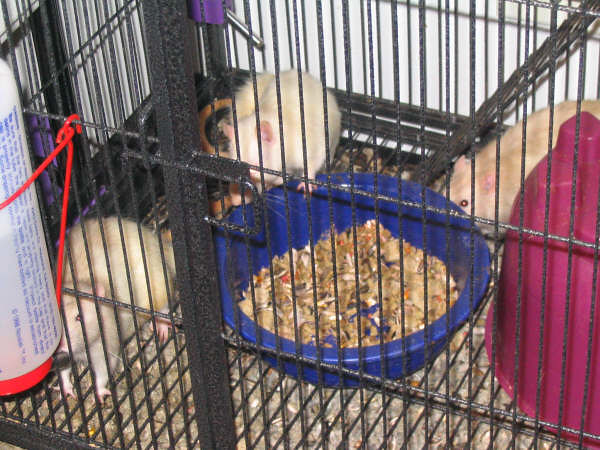This close-up image depicts the inside of a black metal cage housing three light-colored pet rats with a slight brown tint to their fur. Inside the cage, which has a dark powder-coat finish and is constructed of thin vertical bars with a thicker steel outline, the scene is detailed and lively. The central focus is a blue food bowl filled with various kinds of feed, around which two of the rats are gathered, seemingly picking out their preferred pieces in a semicircle. The blue bowl rests on a layer of mulch bedding that spans the bottom of the cage. In the lower left corner, one rat is seen drinking from a clear water bottle with a red wire and cap, attached to the side of the cage. On the right side of the image, there's a burgundy-colored housing structure that might serve dual purposes—either dispensing food or providing a place for the rats to enter and rest. The detailed arrangement also includes a second water bottle with a nozzle and a purple cap, positioned near the other corner.